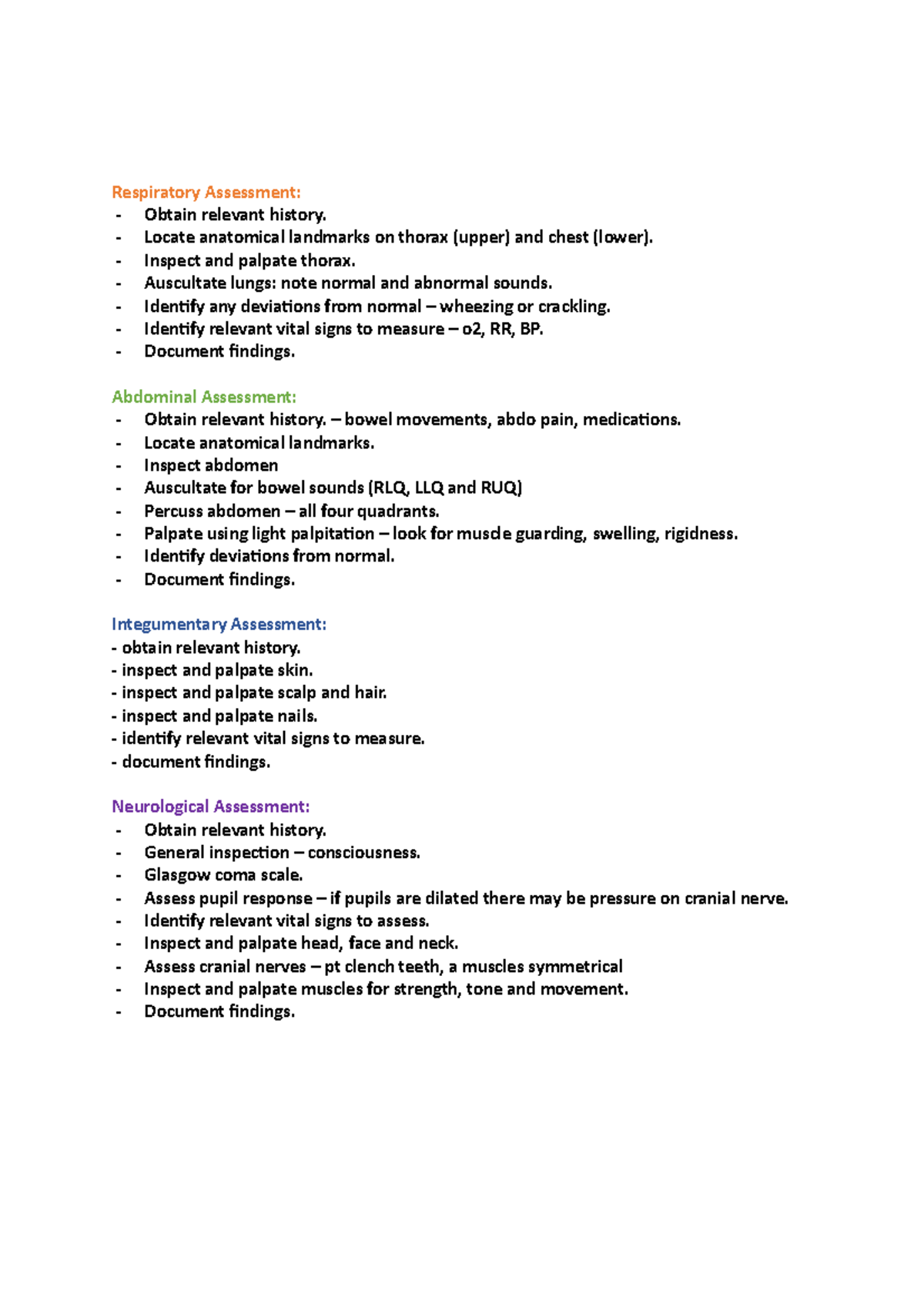**Detailed Caption: Respiratory, Abdominal, Integumentary, and Neurological Assessment**

This comprehensive screenshot from an unidentified source provides a detailed procedural guide for conducting various clinical assessments:

**Respiratory Assessment:**
1. **Obtain Relevant History:** Gather patient’s medical and symptomatic history related to respiratory health.
2. **Locate Anatomical Landmarks:** Identify key landmarks on the thorax, both upper and lower chest regions.
3. **Inspection and Palpation:** Visually inspect and palpate the thorax.
4. **Auscultation:** Listen to lung sounds using a stethoscope, noting both normal and abnormal sounds such as wheezing or crackling.
5. **Identify Deviations:** Recognize any deviations from normal respiratory patterns.
6. **Vital Signs Measurement:** Measure relevant vital signs, including oxygen saturation (O2), respiratory rate (RR), and blood pressure (BP).
7. **Documentation:** Record all findings meticulously.

**Abdominal Assessment:**
1. **Obtain Relevant History:** Record patient’s history regarding bowel movements, abdominal pain, and medications.
2. **Locate Anatomical Landmarks:** Identify key landmarks on the abdomen.
3. **Inspection:** Visually inspect the abdomen.
4. **Auscultation:** Listen for bowel sounds in all four quadrants (right lower quadrant, left lower quadrant, right upper quadrant, and left upper quadrant).
5. **Percussion:** Perform percussion across all four quadrants to assess underlying structures.
6. **Palpation:** Use light palpation to detect muscle guarding, swelling, or rigidity.
7. **Identify Deviations:** Note any abnormalities from the typical abdominal presentation.
8. **Documentation:** Meticulously document all findings from the assessment.

**Integumentary Assessment:**
1. **Obtain Relevant History:** Collect patient history regarding skin, scalp, and hair health.
2. **Inspection and Palpation:** Conduct thorough inspection and palpation of the skin, scalp, hair, and nails.
3. **Vital Signs Measurement:** Measure pertinent vital signs related to integumentary health.
4. **Documentation:** Record the observations and findings in detail.

**Neurological Assessment:**
1. **Obtain Relevant History:** Gather patient’s neurological history.
2. **General Inspection:** Assess general neurological status and level of consciousness using the Glasgow Coma Scale.
3. **Pupil Response:** Evaluate pupil response; note dilations that may indicate pressure on the cranial nerve.
4. **Vital Signs Assessment:** Measure relevant neurological vital signs.
5. **Inspection and Palpation:** Inspect and palpate the head, face, and neck.
6. **Cranial Nerves Assessment:** Assess cranial nerves, including muscle symmetry and strength.
7. **Muscle Assessment:** Check muscles for strength, tone, and movement.
8. **Documentation:** Accurately document all neurological findings.

Each step within these assessment categories is essential for a thorough patient evaluation and contributes significantly to accurate diagnosis and treatment planning.